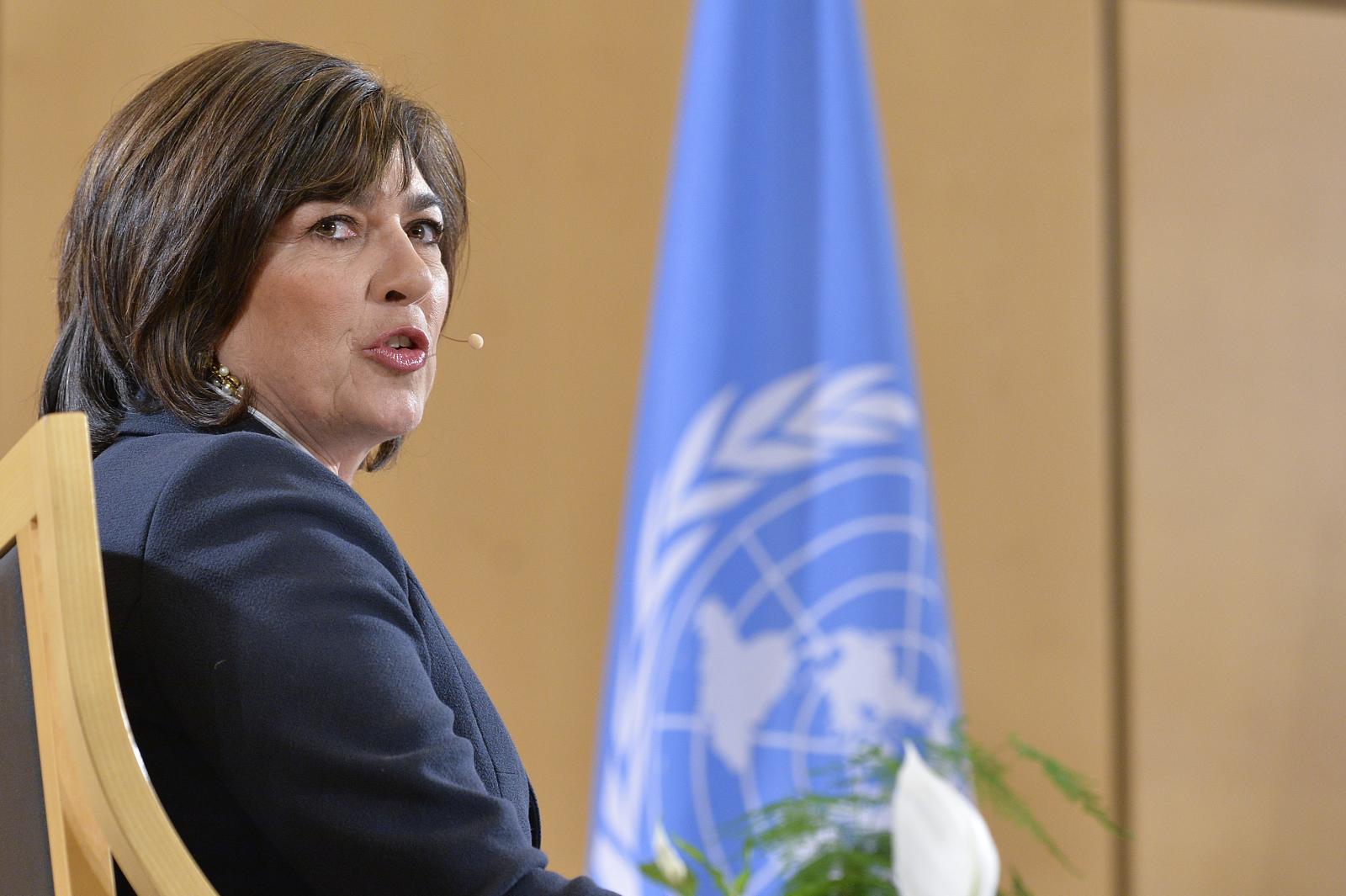A mid-aged woman, possibly in her late 40s to mid-50s, is seated sideways in a light brown wooden chair, gazing directly at the camera. She is dressed in a dark blue suit jacket, and her shoulder-length hair, which features bangs, frames her face. Her dark eyes and eyebrows stand out, and her lips are pursed as if she is in mid-conversation. She is accessorized with earrings that add a touch of elegance. Behind her, a light blue and white flag is prominently displayed in the center of the image. A potted plant with a blossoming white lily adds a natural element to the scene. The background is a neutral light tan wall, providing a subtle contrast to the vivid elements in the foreground.